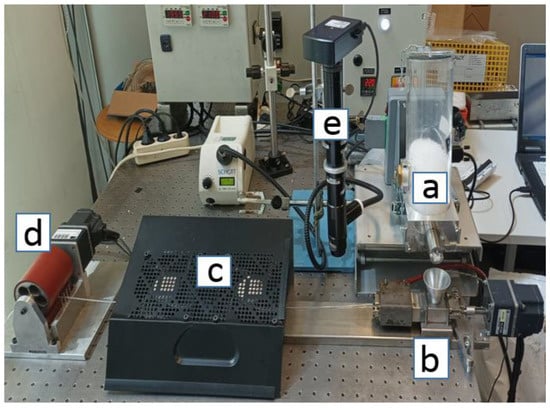The image depicts an old-fashioned desk or worktable cluttered with various pieces of electronic and scientific equipment, each labeled with a letter from A to E. The labels are small, square markers resembling mini post-it notes or tabs. The colors are primarily black, and there is an orangey-red spool on one of the devices, suggesting a possibly outdated setting, maybe from 20 to 30 years ago.

- **Label A:** Marks a clear cylindrical object, possibly a glass beaker or container.
- **Label B:** Identifies a mechanical funnel or apparatus where substances might be dripped.
- **Label C:** Indicates a black rectangular box, potentially a circuit board with a long metal panel attached.
- **Label D:** A cylindrical component, possibly a roller or a drum-like mechanism.
- **Label E:** Points to an elongated electronic component with a part resembling a rectangular battery pack.

The desk also contains numerous wires and plugs, contributing to a somewhat cluttered appearance. Part of a laptop is visible on the right edge of the cropped photo, enhancing the sense of an old, possibly industrial or laboratory setting. The room also appears slightly dingy and dated, adding to the vintage feel of the image.